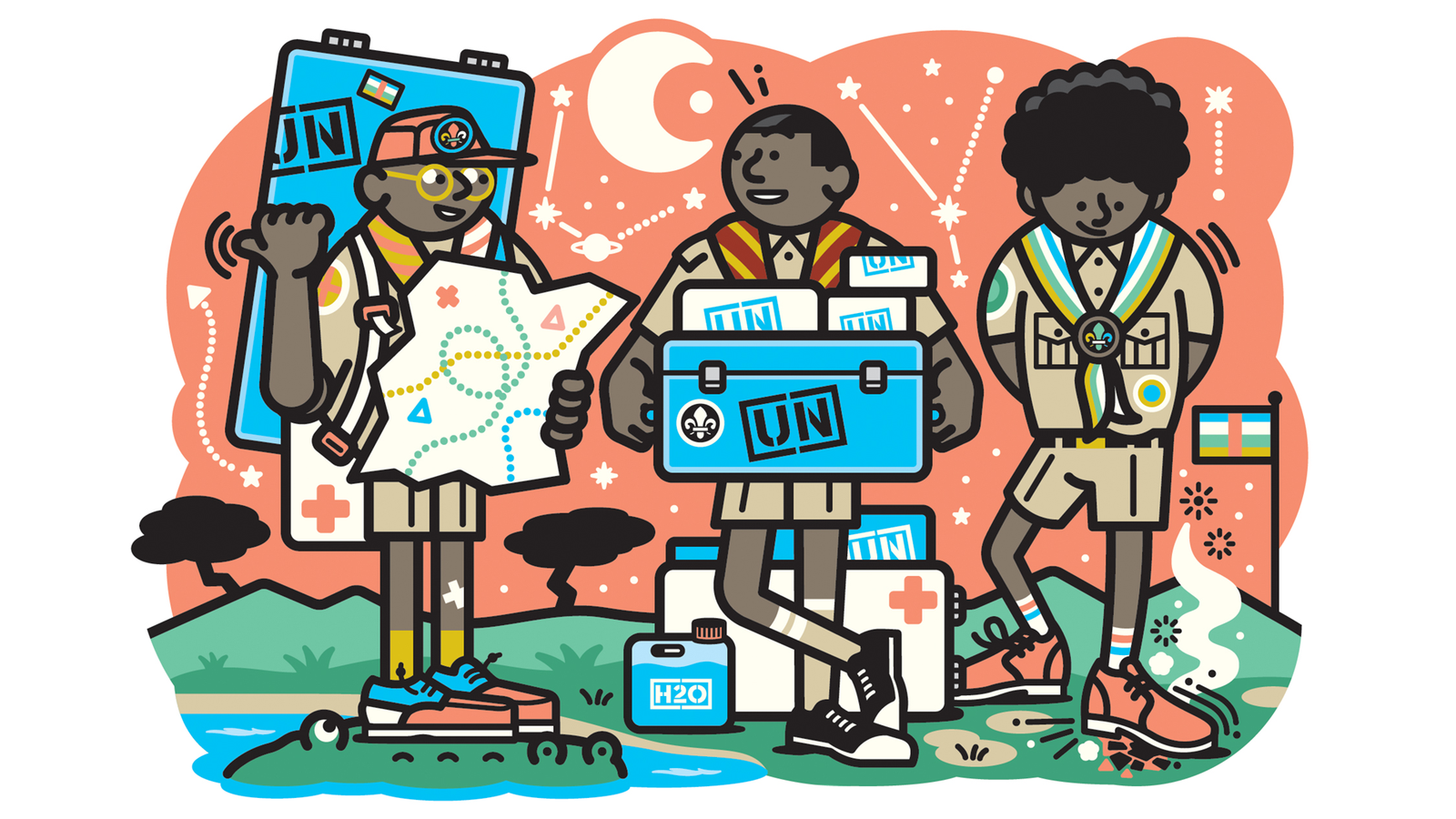The image is an animated illustration depicting three young Black men dressed in Boy Scout uniforms, standing in a vibrant outdoor setting. With a backdrop of peach-colored skies, featuring a crescent moon and constellation outlines, and green hills with trees at the bottom, the scene radiates an adventurous spirit. On the left, the "nerdy" Boy Scout, identifiable by his glasses, holds a map and points to the left. He's standing atop a crocodile's head, with a large blue suitcase on his back stamped with the initials "UN". The middle boy scout holds a blue metal toolbox also marked "UN", along with white packages stacked on top of it bearing the same initials. Behind him is a canister labeled “H2O” and a small white medical kit with a red cross symbol. Lastly, the Boy Scout on the right, characterized by his afro, looks down at the ground as if stomping a bug, with his hands clasped behind his back. All three Scouts are dressed in light brown uniforms with scarves that bear the Boy Scouts symbol on metal sliders, embodying a scene of unity and readiness for an expedition.